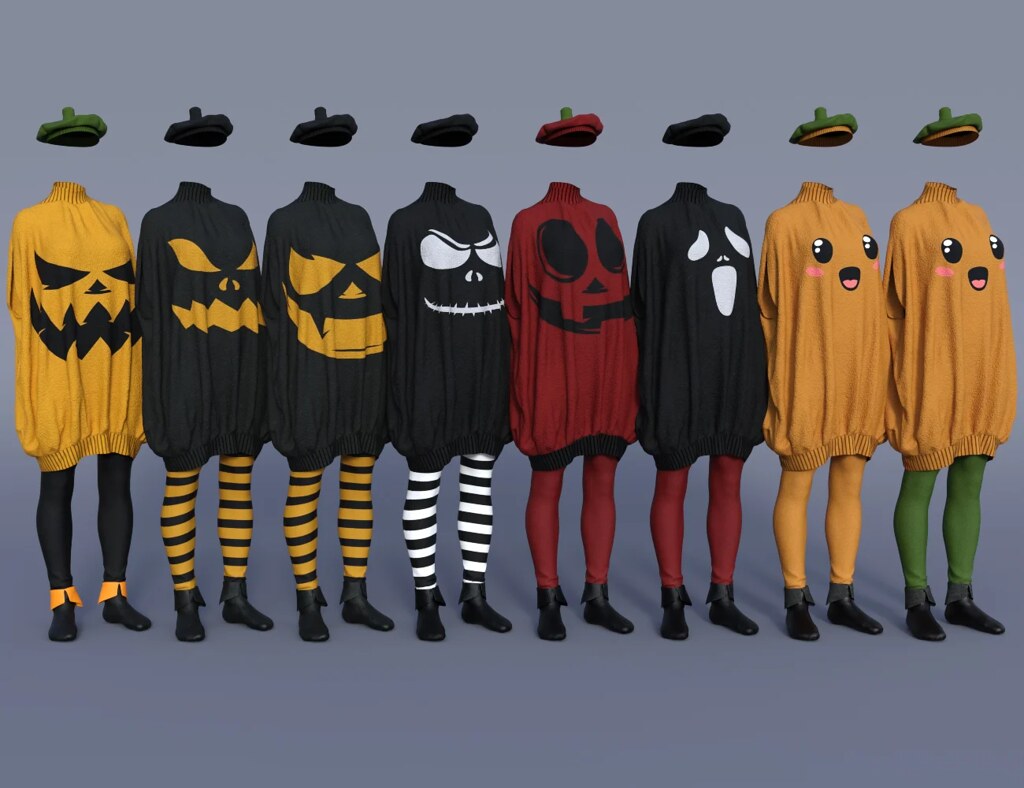The image is a stock-style photograph featuring eight Halloween costumes set against a gray background. The people are standing shoulder to shoulder, with their faces cropped out, creating an illusion of bodies with floating berets above them. Each costume is comprised of a long sweatshirt that falls just above the knee, paired with tights that vary between solid colors and white-and-black stripes, and finished with black boots. The sweatshirts come in different patterns, including three with jack-o’-lantern faces (one orange, two black with orange jack-o’-lanterns), one red with a jack-o'-lantern, one black with a ghost, and others with various spooky characters. These consistent elements—tights, long sweatshirts with Halloween-themed designs, black boots, and berets—highlight the cohesive yet varied style of the costumes.